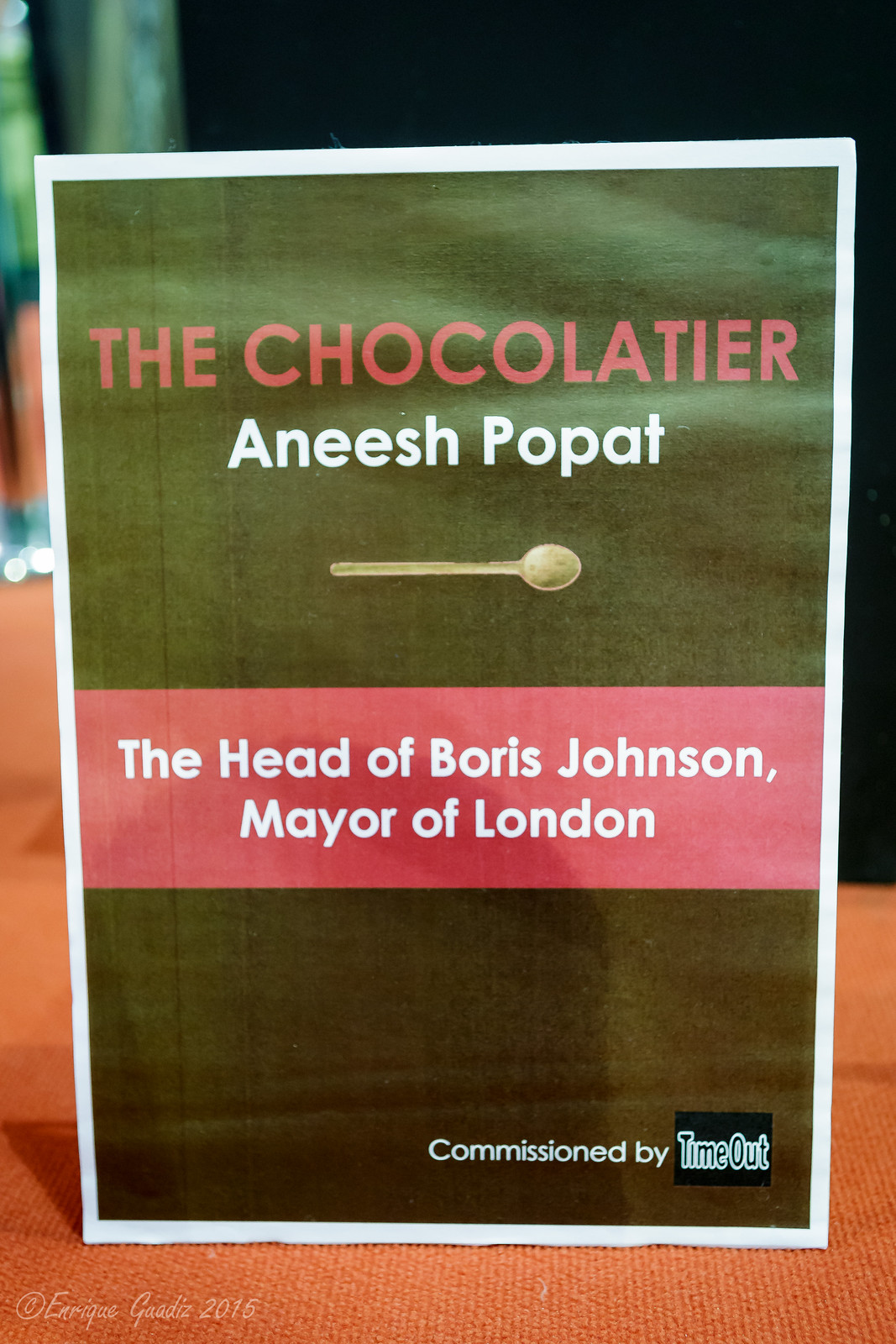This vertical rectangular card features a black background with a white border. At the top, bold red letters spell out "The Chocolate Heir," and directly beneath this, in white letters, is the name "Anish Popat." Below Anish Popat's name, there is an image of a silver spoon. Further down, on a red background with white lettering, it reads "The Head of Boris Johnson, Mayor of London." Finally, at the bottom of the card, it states "Commissioned by Time Out." The card itself rests on an orange background, possibly an orange tablecloth or table, adding a warm contrast to the overall composition.